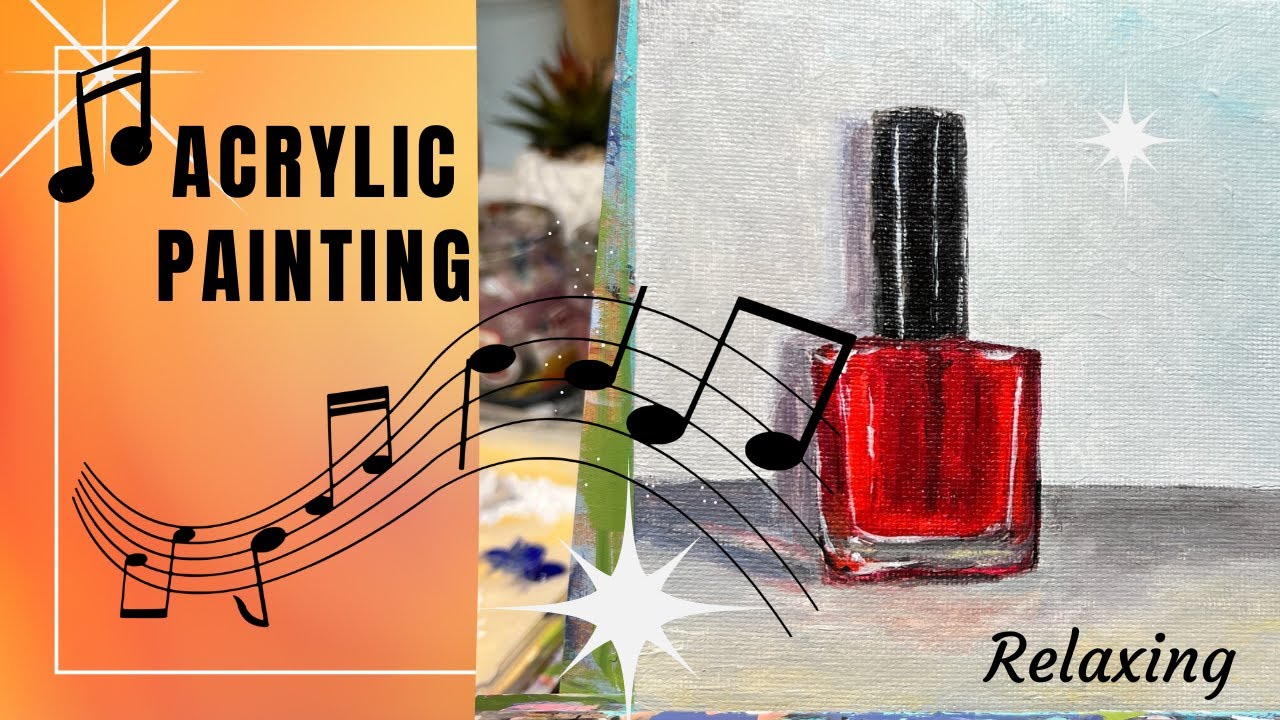The image is split into two distinct sections. The left third, presented as a placard, features a serene ombre orange background that transitions from a darker orange at the bottom to a lighter hue at the top. In black font, it reads "acrylic painting" with a solitary musical note in the upper right corner. A wavy musical staff adorned with notes begins in the lower left of this section, extending seamlessly across into the right two-thirds of the image. The right section, resembling a textured canvas painting, showcases a vividly red bottle of nail polish with a sleek black top. The background seems to be painted with watercolor or pastel techniques, adding to the artistic theme. In the bottom right corner, the word "relaxing" appears in elegant black script. This cohesive blend of visual and textual elements creates a visually appealing and serene composition.